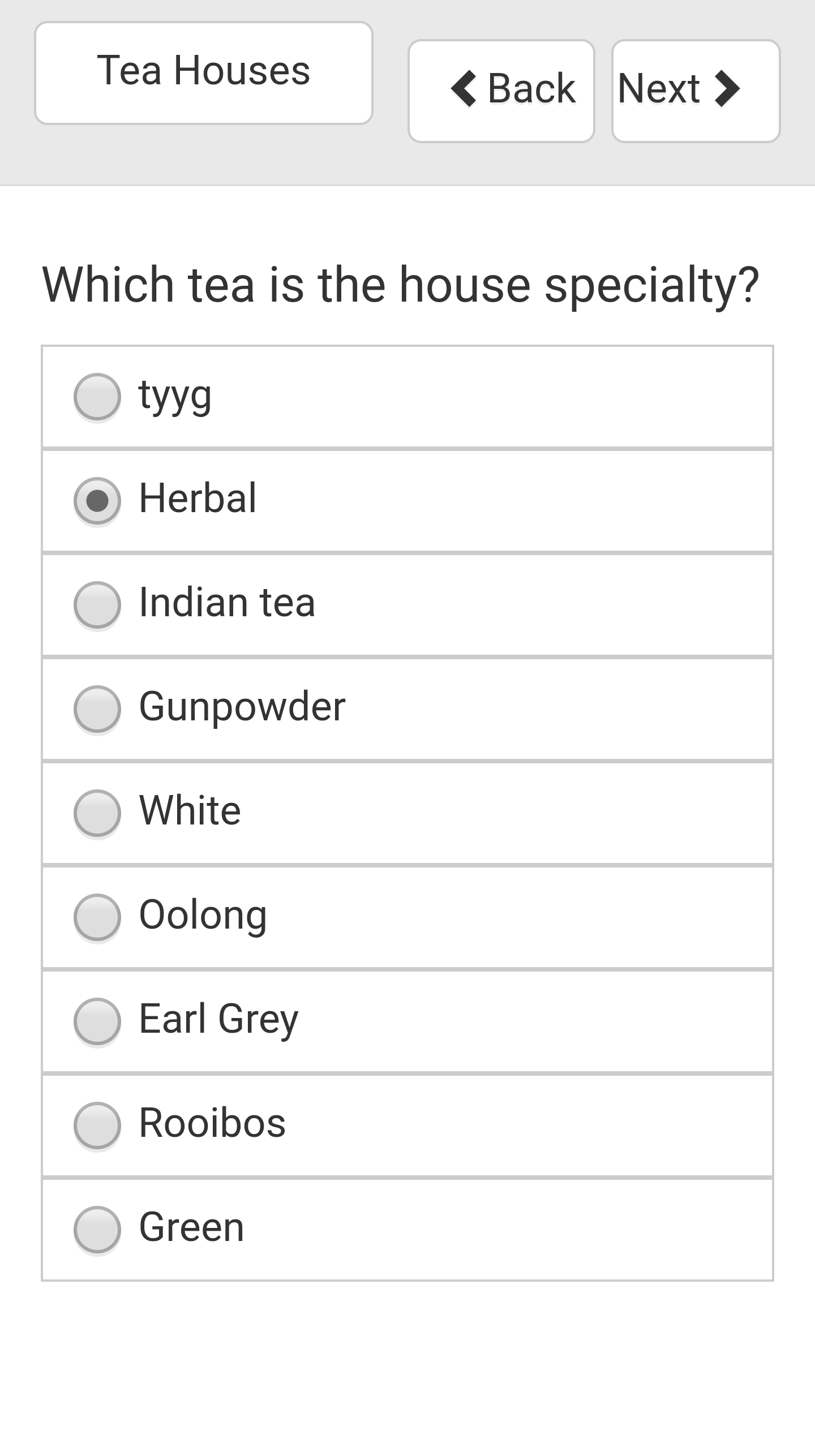The screenshot showcases a section of a website, specifically a partial view of its interface designed for selecting various types of tea. The lilac-colored header at the top features three buttons: "Tea House" on the left, and "Back" and "Next" on the right. Directly beneath this header, a line of text identifies the house specialty tea.

The main section of this screenshot is a neatly arranged list of ten different tea types, each accompanied by a bubble for selection. The list includes the following varieties in descending order:
1. TYYG
2. Herbal (selected)
3. Indian Tea
4. Gunpowder
5. White
6. Oolong
7. Earl Grey
8. Rooibos
9. Green

The list is contained within a box, with each tea type separated by lines. The text is in black, providing a clear contrast against the white background of both the overall page and the individual rows within the box, ensuring readability and a clean, organized appearance.